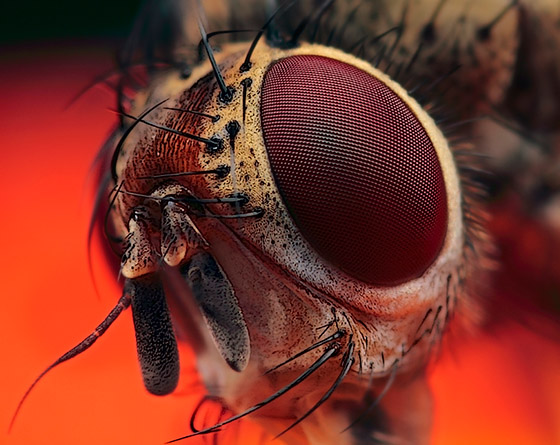This is an extremely close-up, detailed image of a fly's head, with a focus on its large, compounded eye. The eye is a striking red, filled with a grid-like texture. Surrounding the eye, the insect's exoskeleton shines with a metallic gold hue, speckled with black splotches and dotted with black hair-like structures. The fly's head features two antennae positioned where the bridge of a nose would be, and its mouth area is also visible and adorned with black hair-like projections. The background is illuminated with a bright, neon-red light, adding a vivid contrast to the close-up subject. The insect's body, seen in the top right corner, continues the pattern of hairy, gold-colored texture with black markings. The intense detail gives a stark and somewhat unsettling view of the fly, highlighting the intricate and somewhat alien aspects of its anatomy.